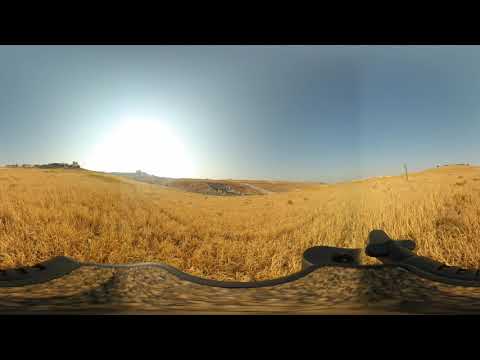The photograph captures a panoramic view of a vast, open yellow wheat field stretching seemingly endlessly under a cloudless, bright blue sky. The image appears slightly warped, hinting at a 360-degree perspective. Black horizontal bars frame the top and bottom of the photograph, suggesting perhaps it was taken through a vehicle's open side or rear. The golden-yellow wheat field extends across the gently rolling hills, occasionally punctuated by distant brown elevations and a few indistinguishable structures in the far background. On the left side of the image, the sun glows brightly near the horizon, casting a serene light over the endless expanse of prairie-like terrain.